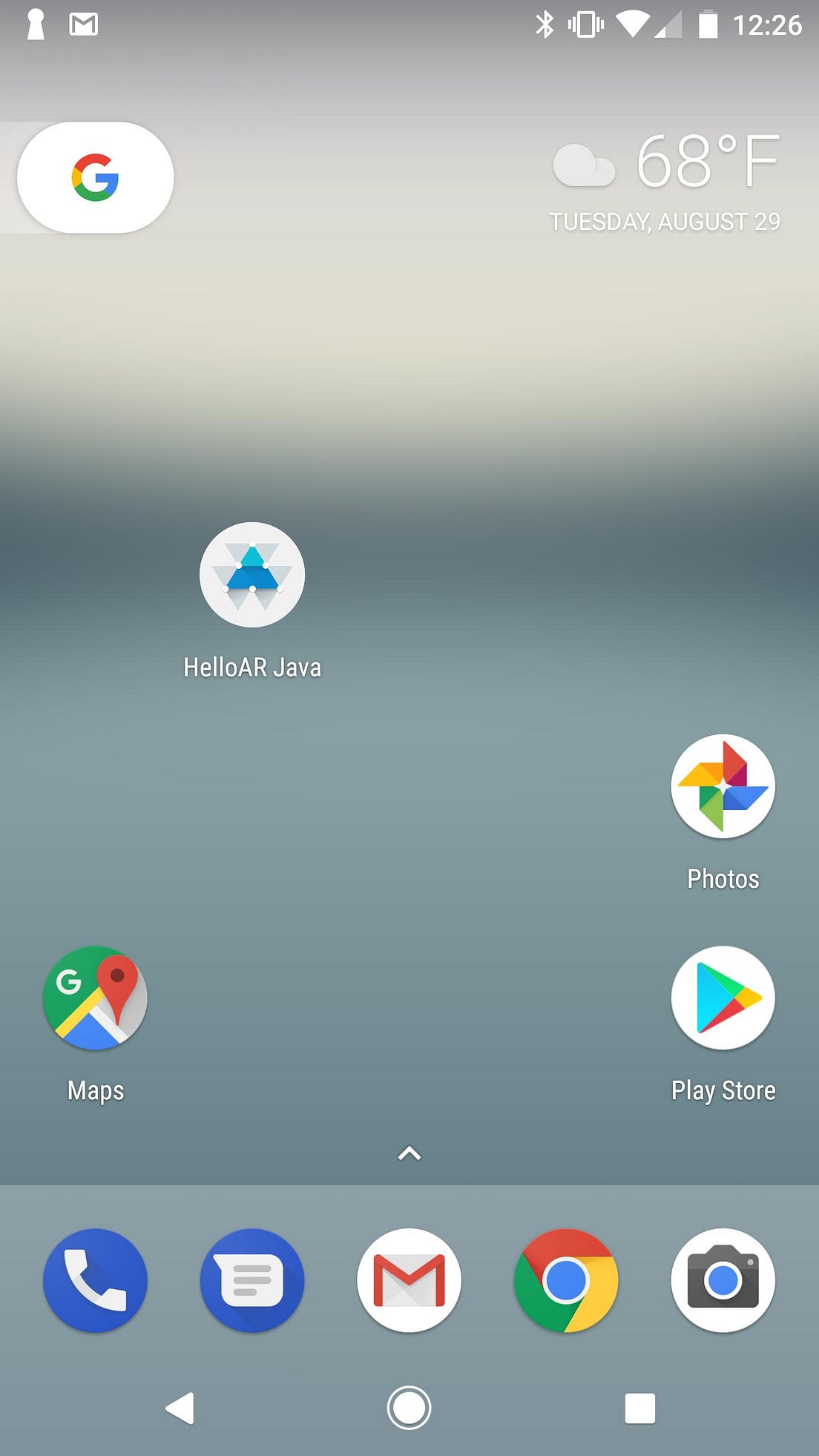The image depicts a smartphone home screen with a gray background at the top, featuring several white icons. The first icon resembles a small person, followed by a white box with a gray "M". There is also the time displayed as 12:26, along with the battery indicator. Below these icons is a semi-circle in a very light gray color.

The white background houses the colorful Google "G" logo in red, yellow, green, and blue. Adjacent to this is a light gray cloud icon displaying "68 degrees Fahrenheit" and the date "Tuesday, August 29". Below, there is a white circle featuring a cluster of three small blue circles with gray points radiating out, labeled "Helio" or "Java" in gray text.

Another circle, green on the left with a white "G" and a yellow stripe, points towards the gray area with a small red pointer, labeled as "Maps" with a white line in blue. Additionally, there is a circle resembling a pinwheel in red, blue, green, and yellow, labeled "Photos". 

Next to it is a white background with a blue, yellow, and red triangle labeled "Play Store", next to a small upward arrow. Following this section, there is a slightly lighter gray block containing several more icons: a blue circle with a white phone, another blue circle with a piece of paper, a white circle with a gray envelope marked with a red "M", followed by the Chrome insignia in red, yellow, green, and blue. Next, there is a white circle with a camera icon showing blue in the lens, and finally, a set of navigation icons: a white pointer, a white circle, and a white square.